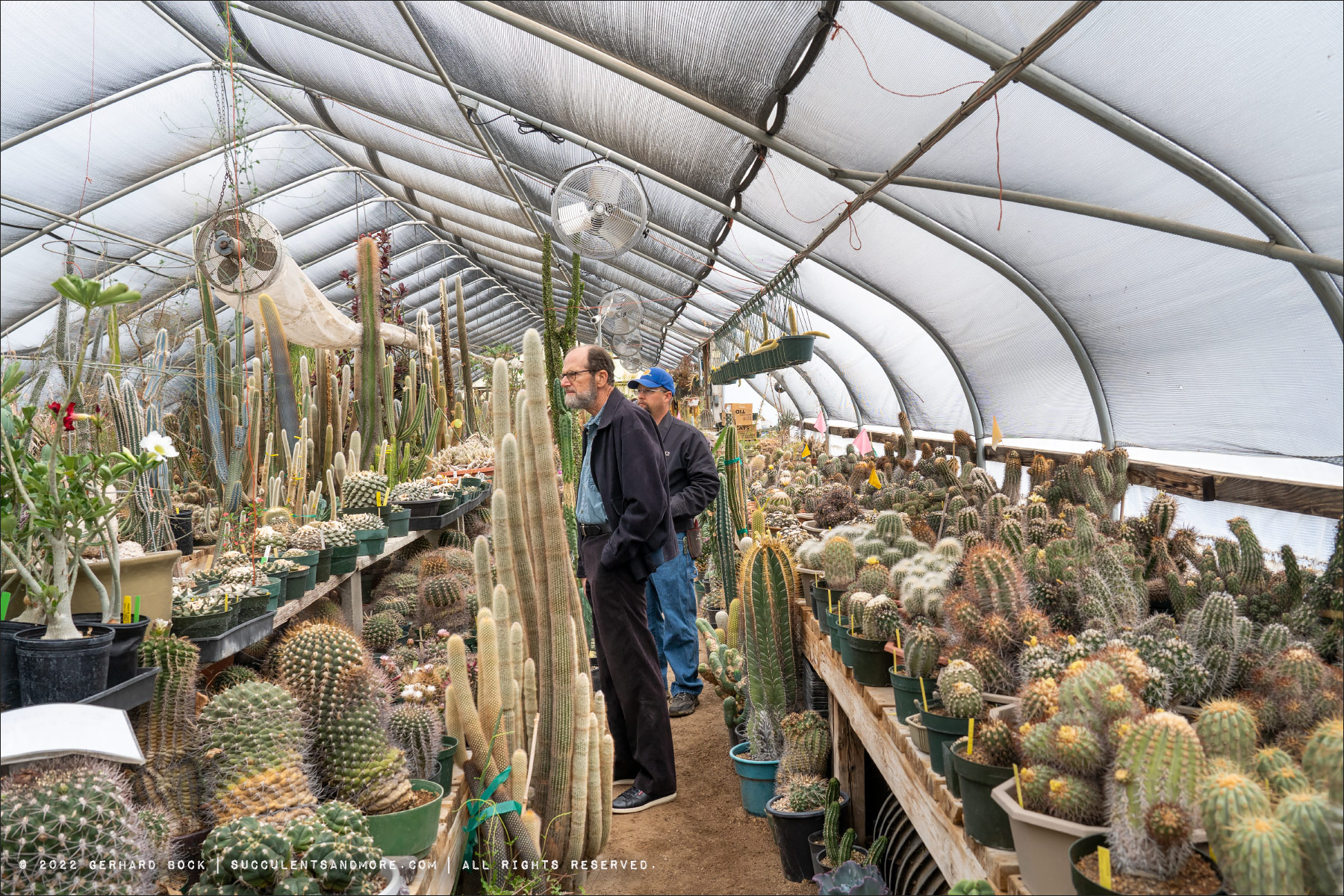The photo captures an expansive greenhouse filled with a diverse array of cacti, ranging from tiny one-inch specimens to towering six-foot-tall plants. The greenhouse features narrow walkways, lined with tables and shelves brimming with both small and large cacti, showcasing varieties with red, white, and yellow flowers. The structure has opaque but clear-colored windows forming the roof, and fans are strategically placed throughout, with some connected to tubes, presumably for ventilation or pollen extraction. The path that the two white male figures are on is composed of brown dirt. The gentleman at the forefront has a balding head with salt and pepper hair and beard, dressed in a blue jacket, blue shirt, and dark black pants. The other man, standing just behind him, is sporting a blue baseball cap, a dark blue shirt, and blue jeans. In the lower right part of the image, a Gerhard book is visible. The scene suggests a retail environment where customers must navigate carefully to avoid the cacti's spines.